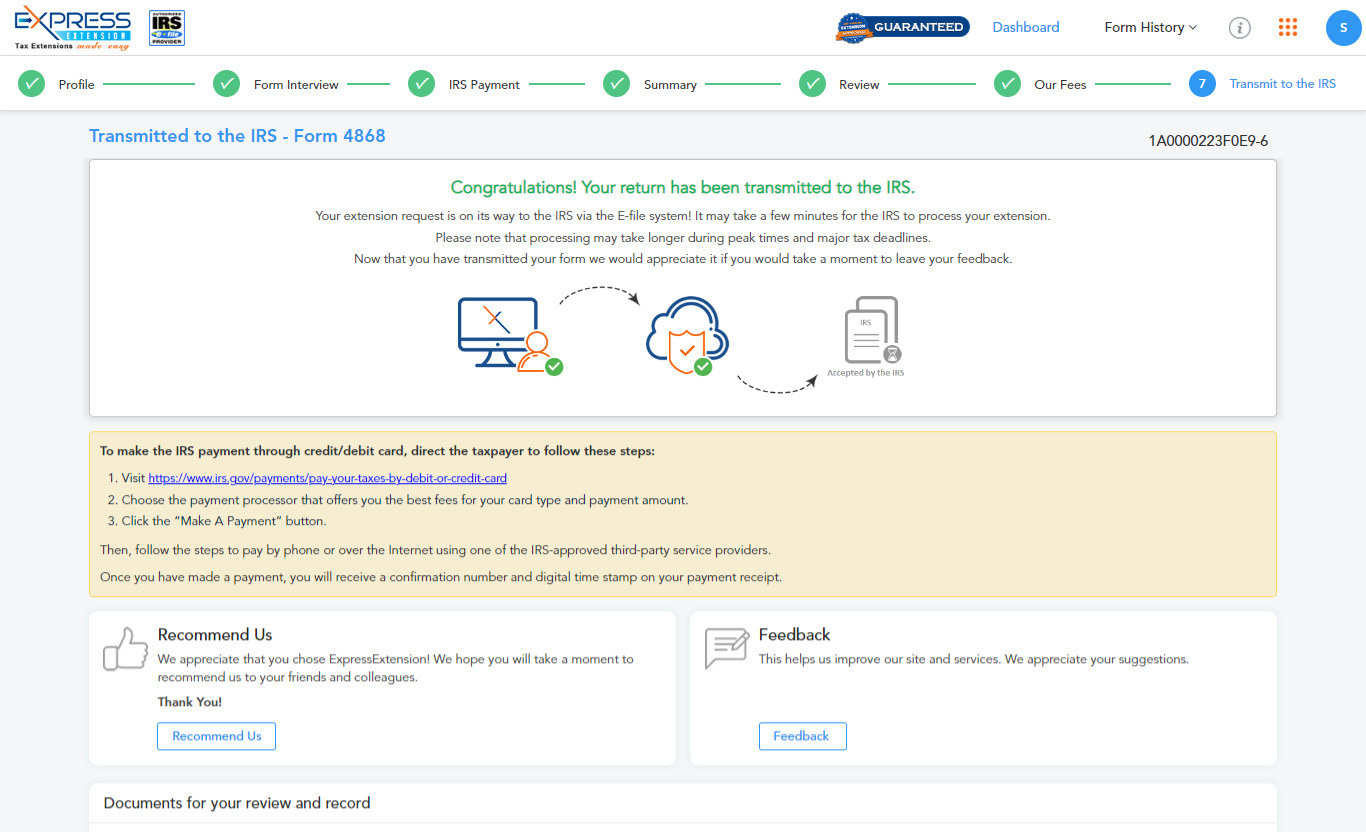A screenshot from the Express Extension website showcases its user interface designed to streamline the tax extension process. At the top of the page, a banner reads "Tax Extension Made Easy" accompanied by an IRS icon, reinforcing the ease of use and official integration with the IRS. A prominent button labeled "Guaranteed" sits across the header, indicative of the service's reliability. A navigation bar features blue text for various sections including "Dashboard," "Form History," and icons such as an information symbol in a gray bubble, nine orange dots arranged in a cube, and an 'S' within a blue circle.

Additional menu options along the top allow users to interact with their "Profile," "Form Interview," "IRS Payment," "Summary," "Review," "Our Fees," and a critical action labeled "Transmit to the IRS" highlighted in blue, marked as step seven in the process. Dominating the center of the screenshot is a congratulatory message: "Congratulations, your return has been transmitted to the IRS." It reassures users that their extension request is currently being processed via the e-file system and advises that this process might experience delays during peak times and major tax deadlines.

In a friendly note, the site also requests user feedback now that the form has been transmitted. To the side, small images offer visual support, enhancing the user experience and engagement.